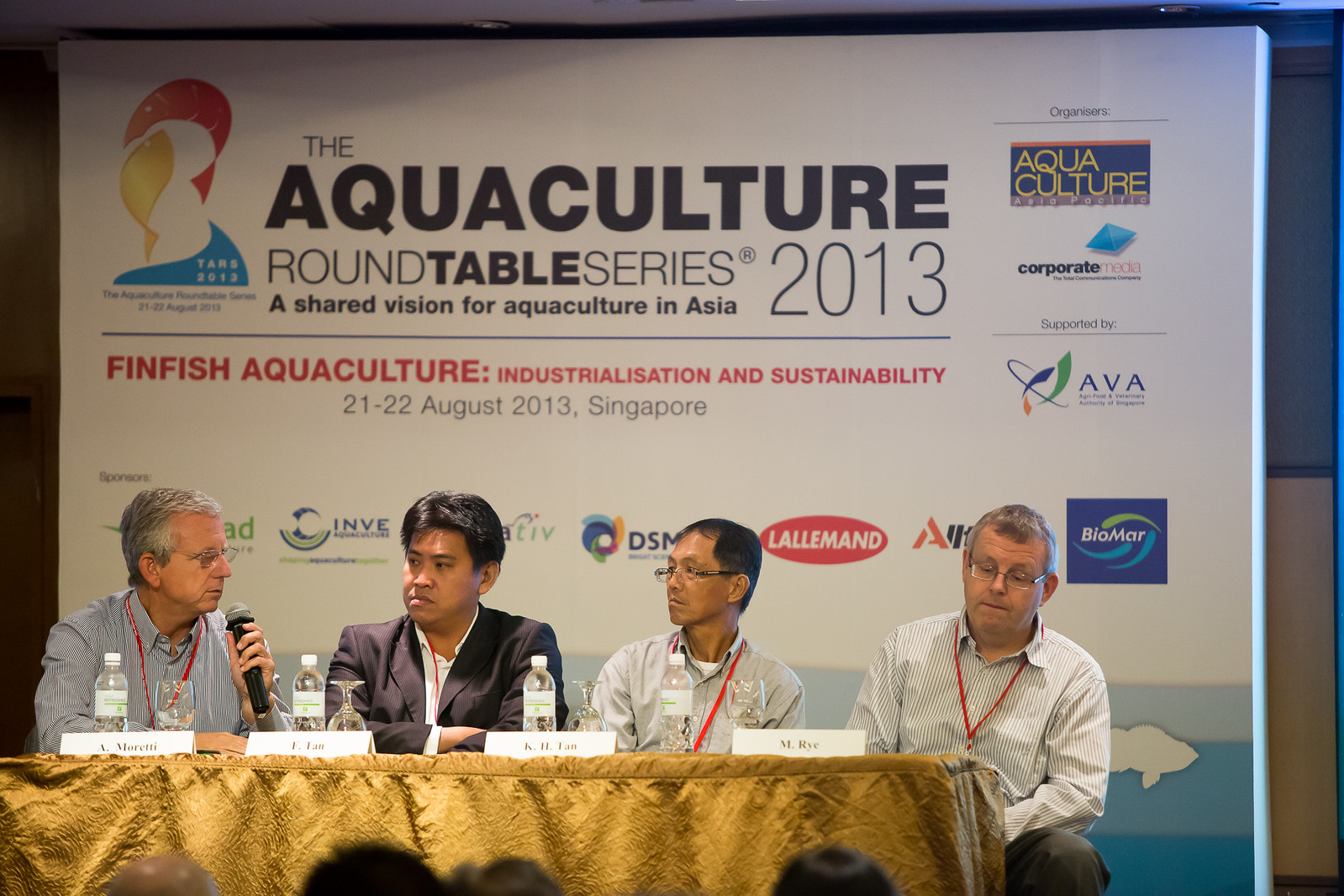This image captures four men seated at a rectangular table, draped with a gold tablecloth, at a conference. They are all wearing business attire, including button-down shirts and lanyards, with one man in a sport coat. Each of them has a nameplate in front of them, reading A. Moretti, E. Lau, K. Ichlan, and M. Rai, along with a water bottle and a glass.

The man on the furthest left is speaking into a microphone, while the two men next to him are attentively looking at him. The man on the far right, however, is gazing off into the distance. Behind them, a large banner reads, "The Aquaculture Roundtable Series 2013, A Shared Vision for Aquaculture in Asia, Finfish Aquaculture Industrialization and Sustainability," and details that the event is held on August 21-22, 2013, in Singapore. The banner, which also features an image of a fish jumping out of the water, includes logos of at least eleven sponsors, like Bayomar, Ava, and Lalamond.